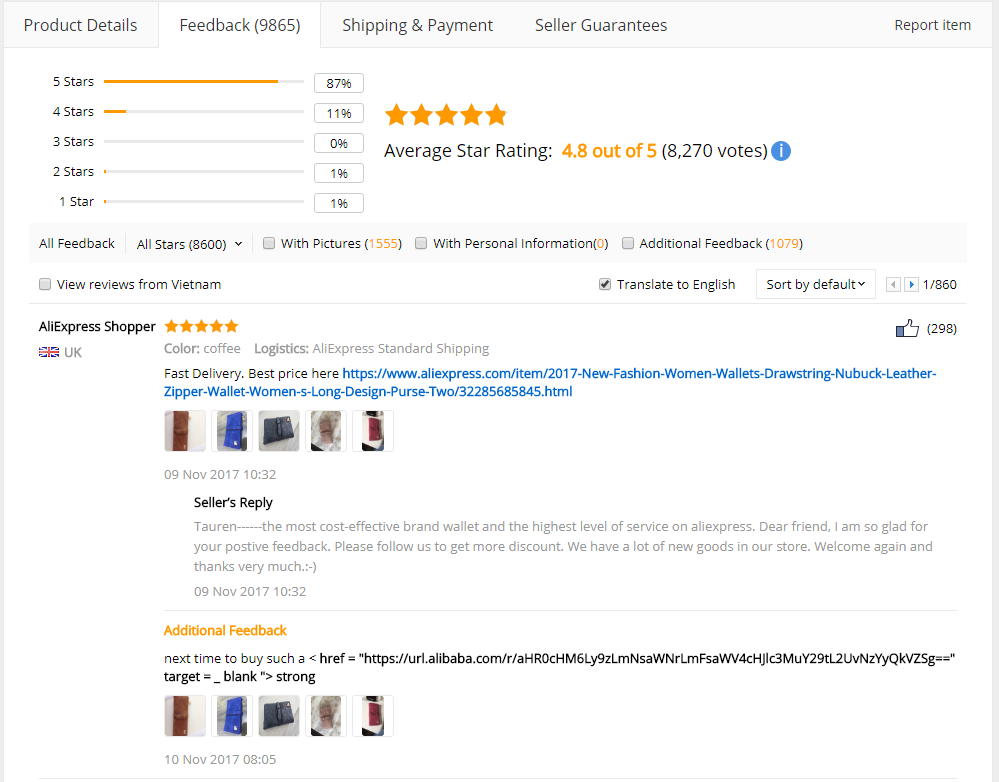This vertical image appears to be a product review page from a shopping website, accessible via computer or smart devices, possibly through an app. The background predominantly features a white screen, bordered by thin gray lines at the top and bottom, with slightly thicker gray lines on the left and right sides.

On the left side of the page, navigation options are visible:
- **Product Details**
- **Feedback** (currently selected)
- **Shipping and Payment**
- **Seller Guarantees**
- **Report Item** (upper right)

User rating statistics are displayed on the left, detailing the distribution of ratings:
- **5 stars: 87%**
- **4 stars: 11%**
- **3 stars: 0%**
- **2 stars: 1%**
- **1 star: 1%**

The product has an overall rating of 4.8 out of 5, based on 8,270 votes. A blue information icon is clickable for more details.

Below the ratings, there are options to filter feedback:
- **All Feedback**
- **All Stars**
- **With Pictures**
- **With Personal Information**
- **Additional Feedback**

Reviews include geographic information, with a section particularly for reviews from Vietnam, translated into English. The default sort order is indicated. Reviews typically include:
- The reviewer's identity (AliExpress shopper)
- The product purchased
- The reviewer's location
- Attached pictures of the product
- Seller's replies

At the bottom of the page, further feedback options are provided.